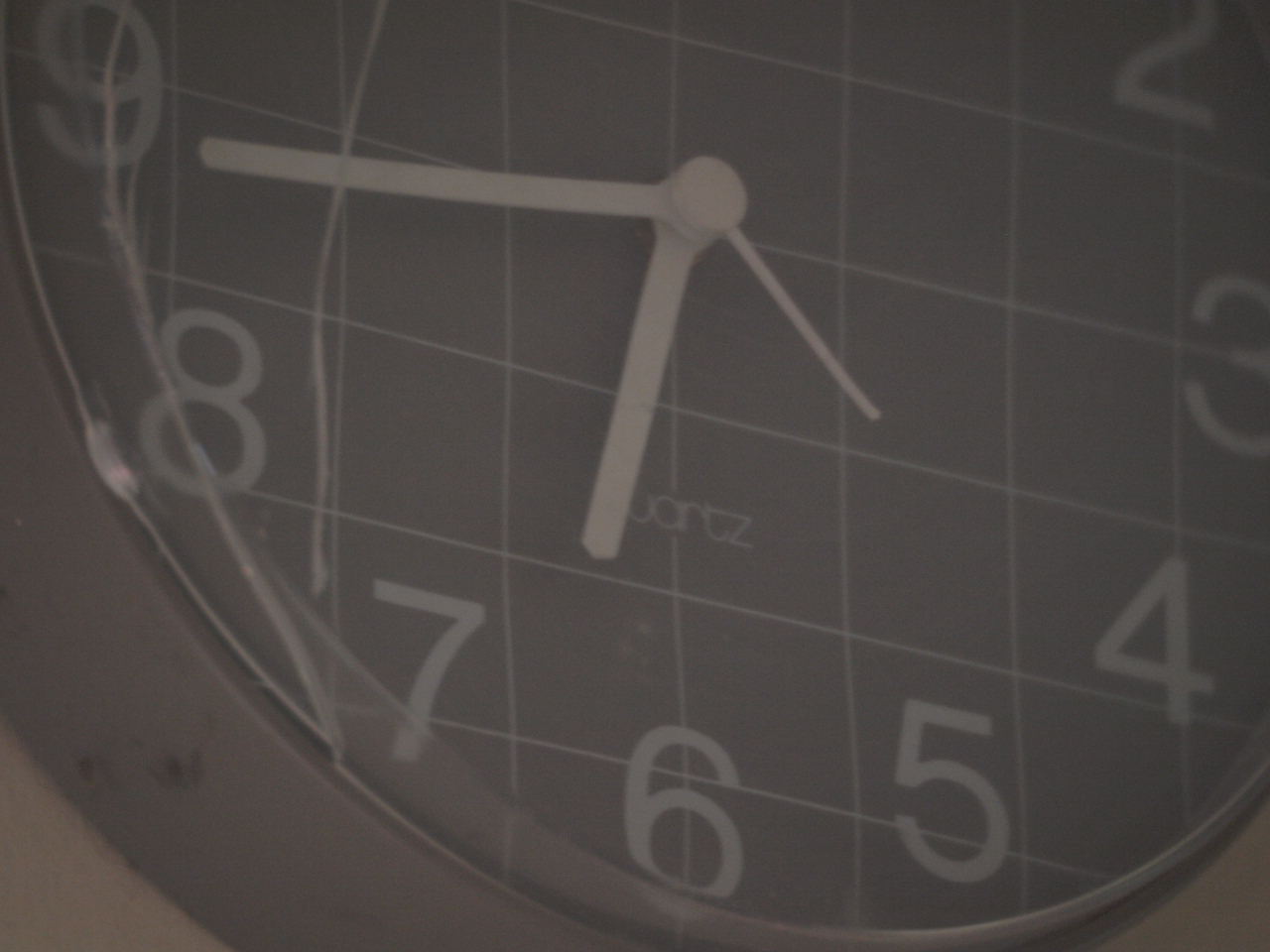A close-up image of a vintage quartz wall clock, taken under very dark conditions, reveals an aged and weathered timepiece. The round, silver-gray bezel encases a dial where the gray background displays a subtle light cross-hatching pattern. The clock features simple, straightforward numerals and old-fashioned, stubby hands for the hours and minutes, along with a short, inexpensive-looking second hand. The word "Quartz" is inscribed in the center. The clock's crystal is visibly cracked, suggesting it has endured some abuse. Additional wear is evident from marks on the bezel, particularly in the lower left corner. The backdrop appears to be a plain wall, emphasizing the clock's utilitarian and vintage aesthetic.